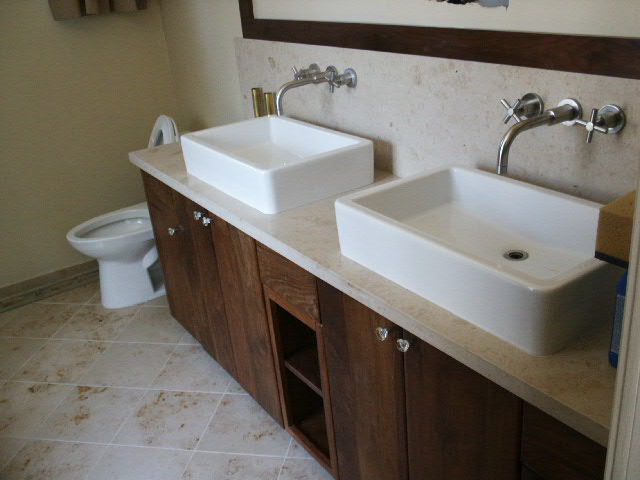This is a detailed photograph of a modern bathroom with a neutral color palette. The focal point of the image is a double vanity on the right-hand side, featuring two rectangular white porcelain vessel sinks mounted on a light beige marble countertop. The countertop extends partially up the wall, merging seamlessly with the backsplash. Each sink is paired with sleek, brushed silver faucets that protrude from the wall above, providing a contemporary touch. 

Above the vanity is a large rectangular mirror framed in wood, although it is not entirely visible in the image. Beneath the sinks, the dark brown wooden cabinetry, adorned with clear crystal knobs, provides ample storage space. The cabinetry's dark hue contrasts with the light theme but complements the overall aesthetic. 

The floor is covered in tan tile arranged in a diamond pattern, accented with dark brown splotches that lend it an organic, somewhat rustic appearance. The tiles create a textured look that adds depth to the otherwise minimalist design.

On the far left side, partially obscured behind the vanity, is a simple white porcelain toilet with both lids up, suggesting recent use. The walls of the bathroom are a soft beige, and the baseboards are a matching tan color, enhancing the room's cohesive and tranquil feel.